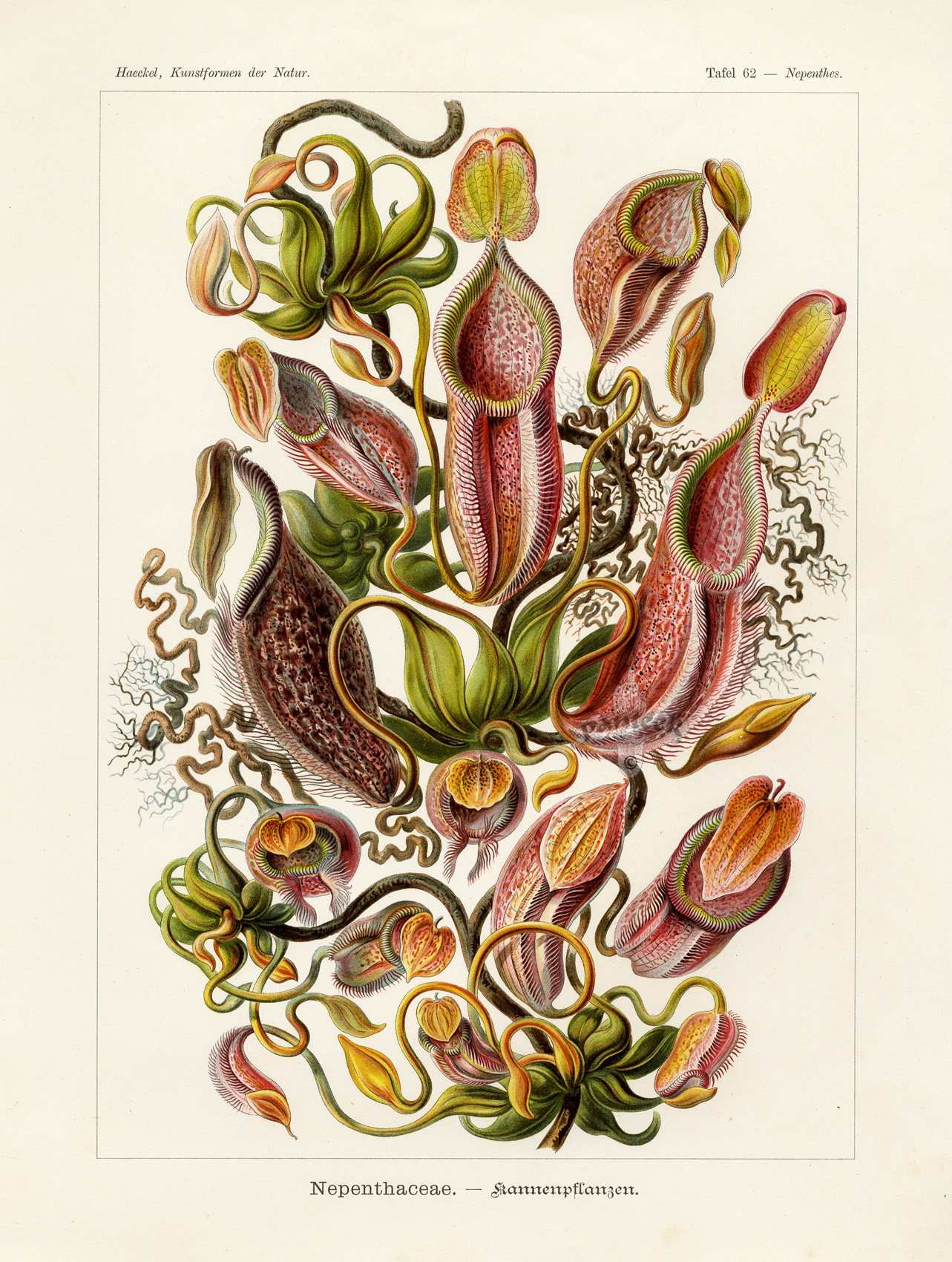This detailed botanical illustration, taken from Haeckel's "Kunstformen der Natur," features diverse and whimsically drawn Nepenthes plants, resembling abstract art. In the top left corner, italic text identifies the source, "Haeckel Kunstformen der Natur," while the top right corner reads "Tafel 62 Nepenthes." At the bottom, the scientific name "Nepenthaceae" is displayed in a Gothic font.

The illustration showcases curvy, cylindrical red flowers with green borders at their tips, reminiscent of open Venus flytraps. These unique blooms vary in their stages of development, starting from small, unbloomed buds to fully bloomed yellow flowers with red bases, interspersed with elongated heart-shaped leaves in orange and green, alongside standard green leaves.

The depiction is busy and organic, with twisting vines and various leaf shapes intertwining, contributing to a visually intricate and somewhat confusing arrangement, making the Nepenthes plant appear both exotic and fantastical.